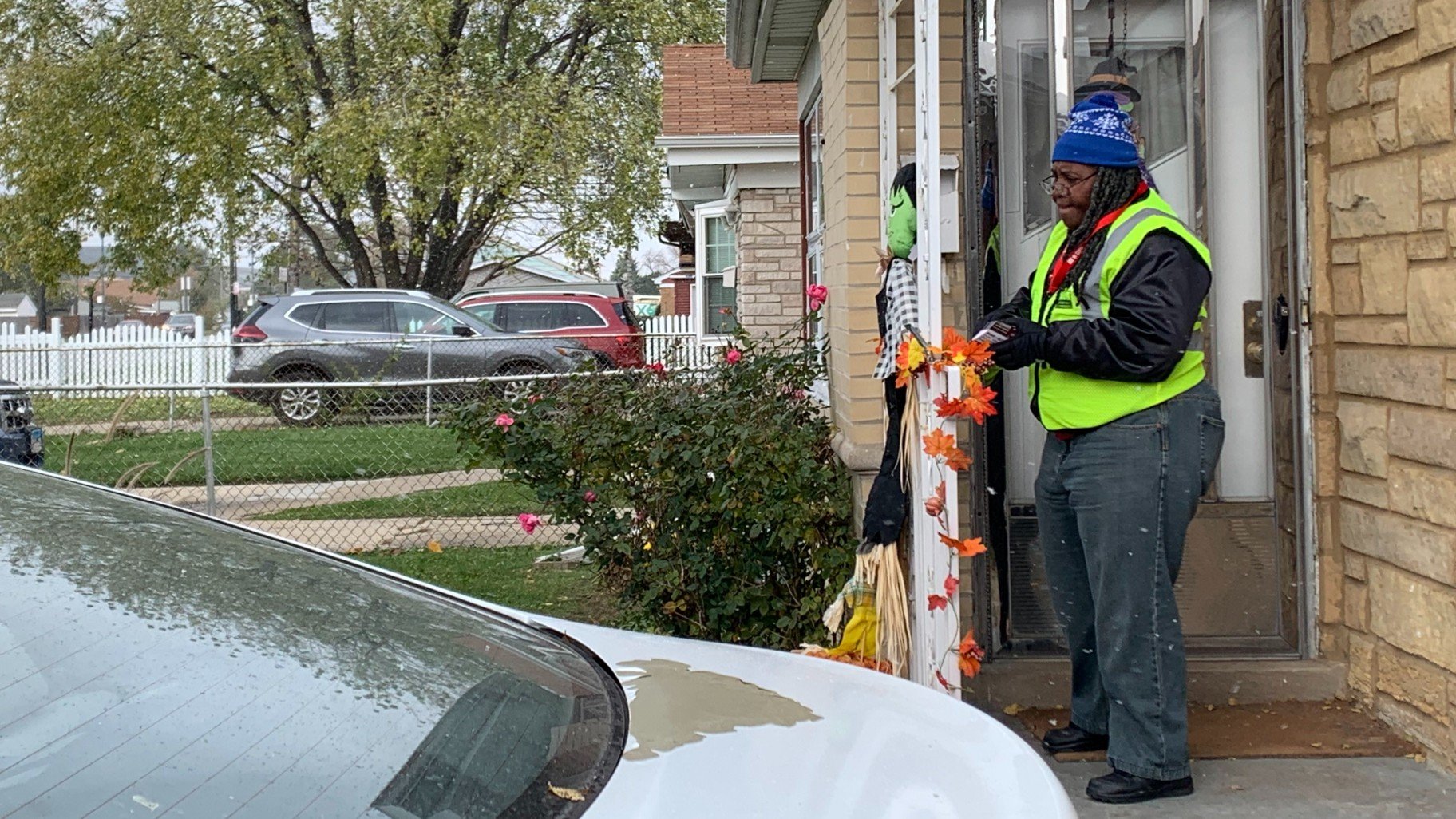The photograph captures an outdoor setting in front of a house with beige stone walls. On the right side, an African American woman stands on the doorstep, facing left. She is wearing a neon green safety vest over a black jacket, gray jeans, and black sneakers. Her attire includes a blue and white knitted beanie with snowflakes and long black dreadlocks. The woman appears to be a government worker and is seen arranging orange leaf Halloween decorations on a white railing by the door.

A white car is partially visible on the left side of the image, with its back end and a small bush with pink flowers beside it. Additional cars and houses with red roofs, chain link fences, and green lawns are visible in the background. A large tree rises behind these houses. The house's entrance features a brown rectangular doormat. The scene is defined by a mix of residential elements: vehicles, fences, and seasonal decor, painting a vivid picture of a neighborhood during a festive season.